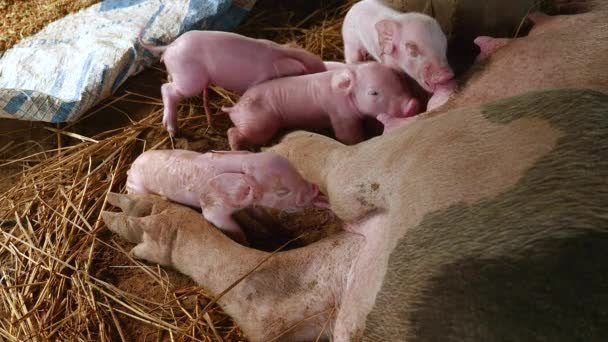This image captures a tender scene of four newborn piglets nursing from their mother. The piglets, mostly light pink, nestle against their mother's body, which is predominantly light brown with darker brown and black patches. One piglet appears slightly whiter than the rest, situated near the top. The mother pig lies on a bed of dry, gray and yellow hay, her back legs stretched out, with one piglet tucked between them and the other three closer to her upper body. Though her face is not visible, her nurturing presence is evident as the piglets feed. In the upper left corner, a white package with blue stripes can be seen, adding a touch of curiosity to the otherwise earthy farming scene. This heartwarming image, marked by the contrast of pinks and browns against the rustic straw, would be an ideal fit for a personal or farm blog, capturing a simple yet beautiful moment of life on the farm.